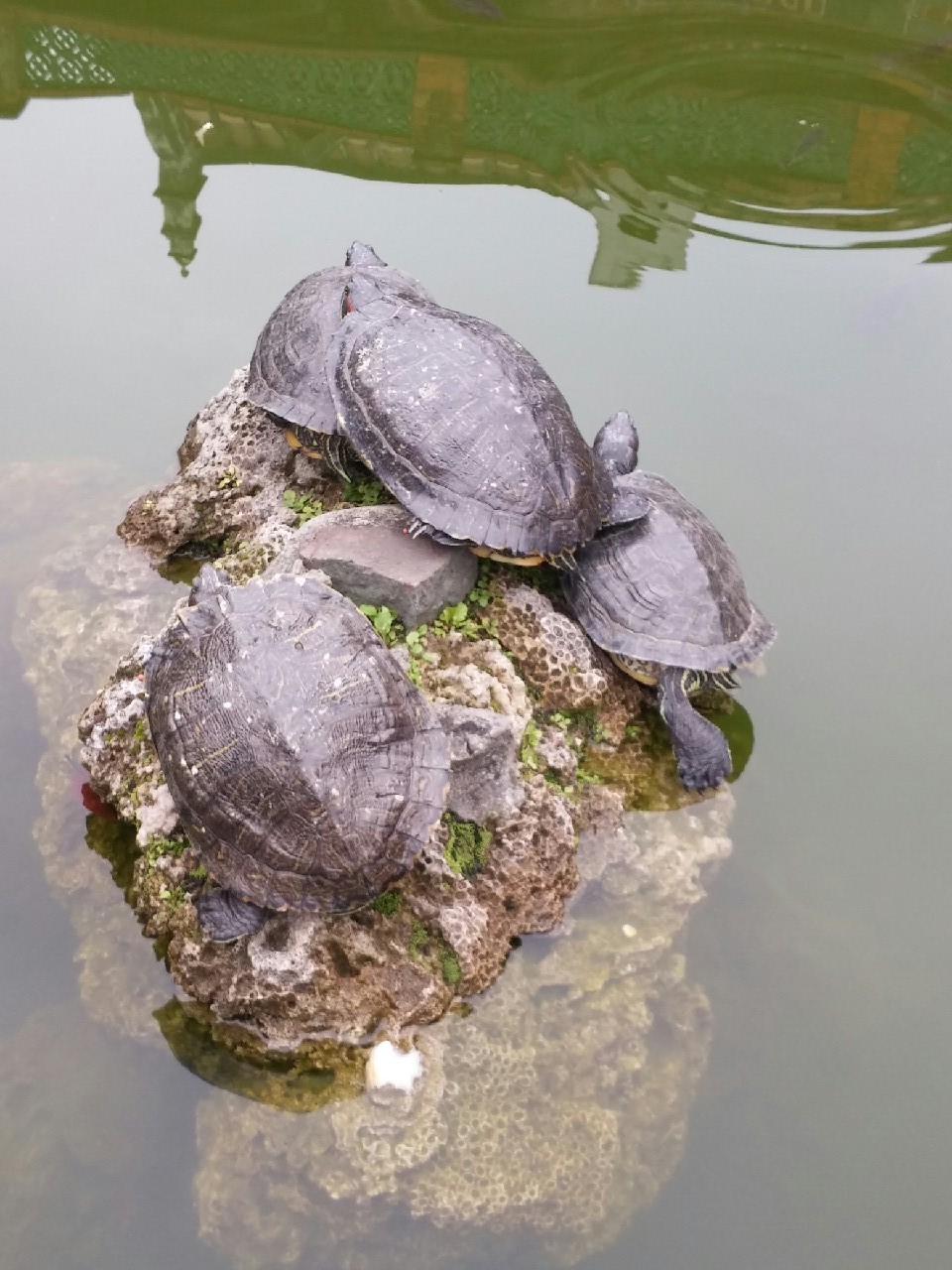In this captivating photograph, four sizable turtles with dark brown, shiny shells are leisurely basking in the sun on a rough, coral-like rock protruding from murky, greenish water, possibly a pond or swamp. The rock transitions from a pinkish-brown hue above the water to a whiter shade below, with some green growth adorning its surface. The turtles, all facing away, display their legs and shells in striking detail. The water is slightly disturbed, forming concentric rings, and reflects a structure with green and red elements, as well as a fence-like object in the background. This serene scene invites a closer inspection of the turtles’ peaceful sunbathing amid their natural, reflective surroundings.